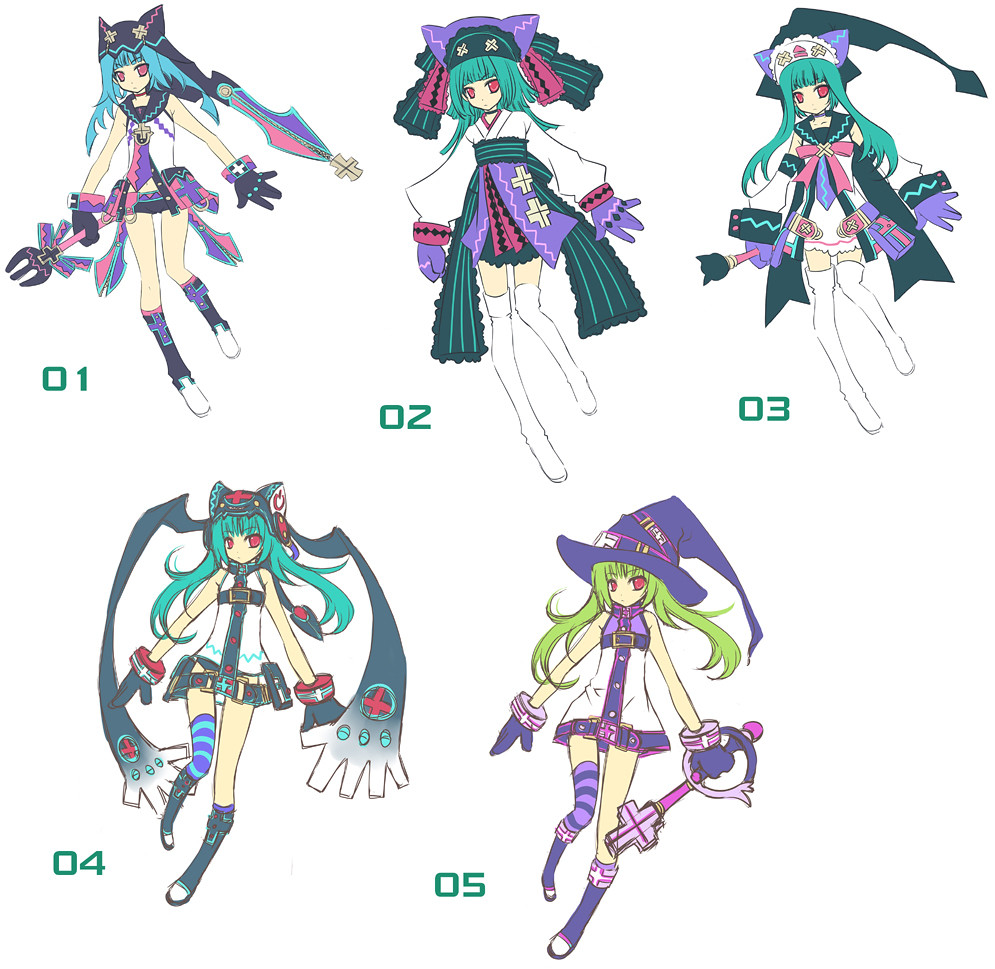The image is a square-shaped illustration set against a completely white background, showcasing five different sketches of a young female anime character. The sketches, numbered 01 to 05 in dark green on the lower left corner, are arranged with three on the top row and two on the bottom row. Each drawing depicts the character with various outfits and accessories. The character consistently has red eyes and varying shades of green hair, from aqua to teal, with one sporting lime green. She carries a pink pitchfork in her right hand across all sketches. Her hair features a distinct blade-like strand ending in a cross, colored in purple and pink. Each character is adorned with hats, some with cat ear shapes, and one with a witch-style hat. The color schemes blend greens, purples, pinks, and blues. Notably, the top left character has shorter, aqua-colored hair, the top middle and bottom left characters have long strands hanging off their hats, and the outfits share a thematic mix of gray-blue, light pink, and purple, accented with teal or blue. The top left, top right, and bottom right characters hold scepters, and the bottom right character uniquely holds a key with a cross in her left hand.